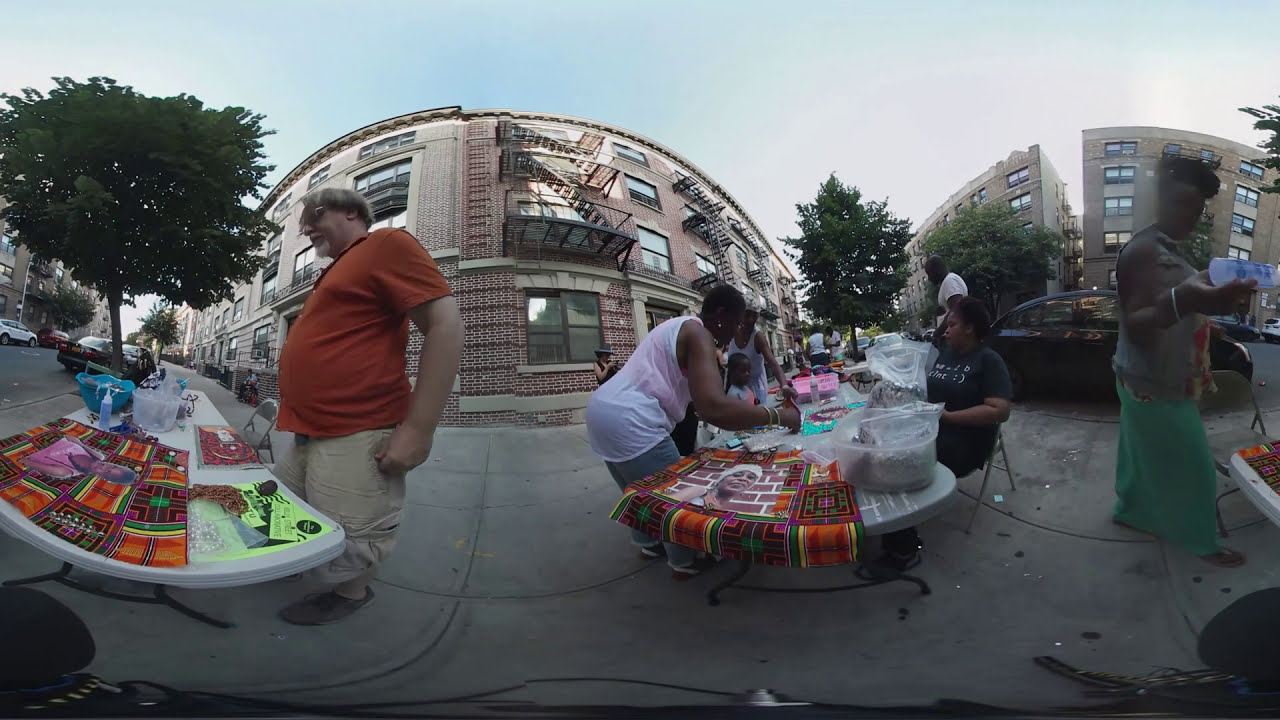The photograph captures a vibrant, outdoor sidewalk market bustling with activity under a clear blue sky adorned with wispy white clouds. Spanning the frame, the market is set against a backdrop of brick apartment buildings featuring black railings and fire escapes. The street is lined with parked cars, including a white SUV and several black vehicles.

Front and center, a man in an orange short-sleeved t-shirt and khaki pants stands behind a white plastic table adorned with a colorful array of wares, including an orange quilt, various bowls, and a spray bottle with purple liquid.

To the left, another vendor, a seated African-American woman in a dark short-sleeved shirt, tends to her table, which is covered in African-patterned fabric and displays an array of jewelry. Beside her, a standing woman leans over the table, dressed in a white shirt and gray pants, seemingly absorbed in examining the items.

On the right side of the image stands a woman in a long green skirt and a blue denim jacket, holding a bottle and looking towards the camera. The tables around her display more colorful fabrics and products, with other vendors and customers, including a small girl, engaging in lively exchanges. 

The sidewalk is dotted with fold-out chairs and bustling with the activity of both standing and seated individuals, all contributing to the lively, urban street market scene.